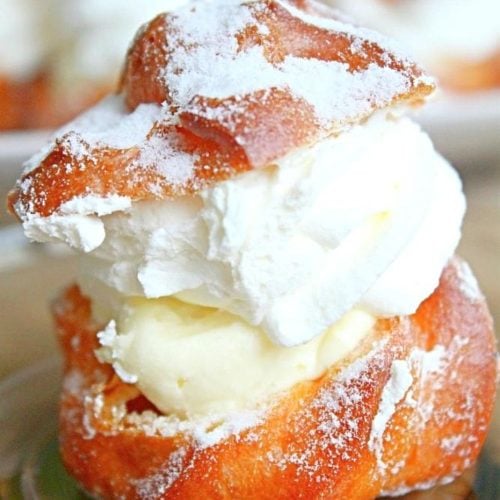An up-close, detailed photograph captures a decadent dessert, likely a cream puff, with two golden brown pastry halves dusted with powdered sugar. The bottom half cradles a creamy, pale yellow scoop resembling vanilla ice cream, topped by an even larger, fluffy dollop of whipped cream. The dessert, taking center stage of the image, sits elegantly on a clear glass plate. The backdrop of the photo is blurred, hinting at a restaurant or bakery setting with indistinct colors and shapes, keeping the focus on the sumptuous pastry.